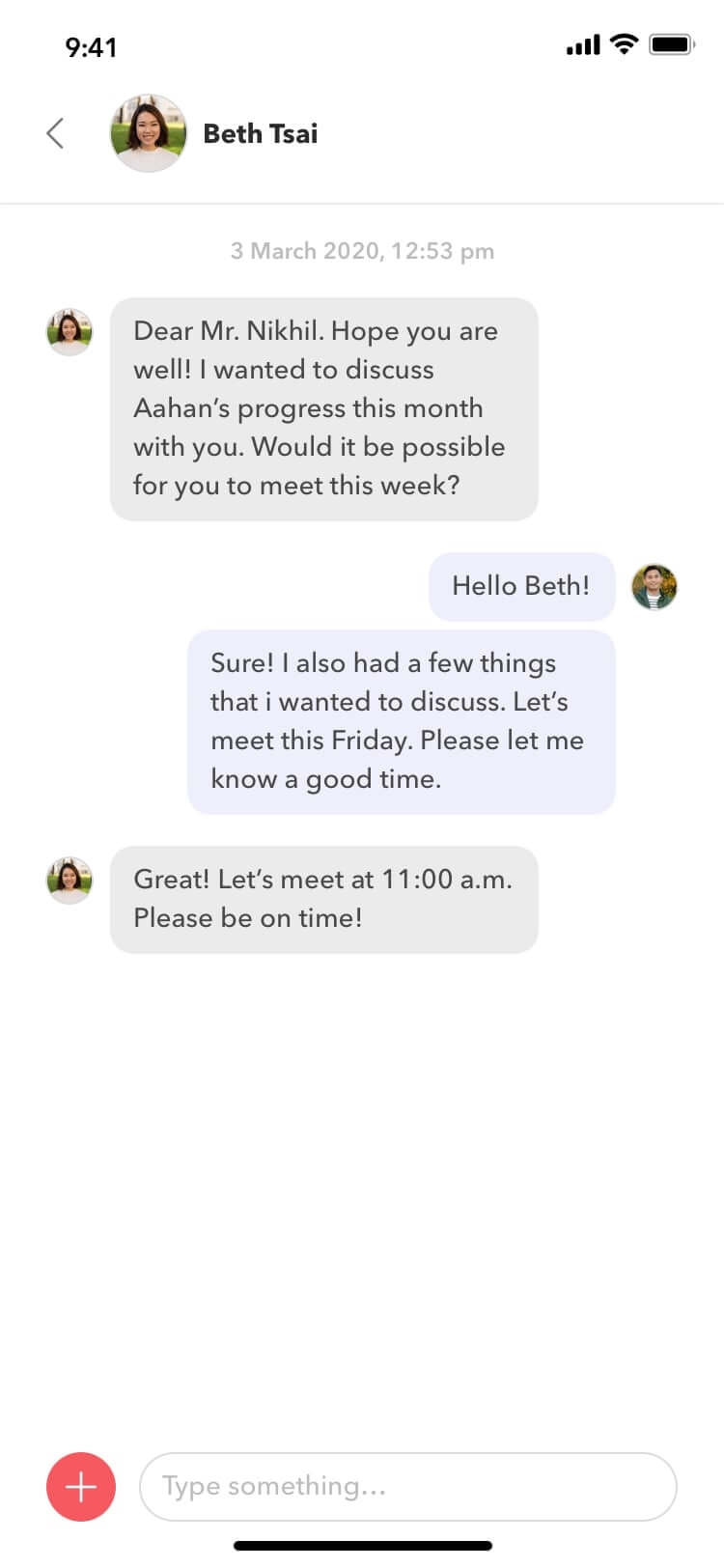The screenshot captures a chat interface on an iPhone at 9:41 AM, as indicated in the upper-left corner of the screen. To its right, a series of icons display complete network and Wi-Fi connectivity alongside a fully charged battery symbol. The top portion showcases a chat application, beginning with a back arrow followed by a profile picture of a woman labeled "Beth Tasami." Below her name, a timestamp reads "3rd March, 2020, 12:53 PM" alongside the onset of a chat thread.

The dialogue begins with Beth Tasami's message: "Dear Mr. Nick, hope you are well. I want to discuss Anne's progress this month with you. Will it be possible for you to meet this week?" The interface also features a plus icon encased in a red circle for additional functionality, located at the bottom left. Beside it lies a search box with rounded corners labeled with placeholder text: "Type something..." A sleek black horizontal line with rounded corners demarcates the input area for new messages.

The conversation continues with a response from Mr. Nick: "Hello, Beth! Sure! I also had a few things I want to discuss. Let's meet this Friday. Please let me know a good time." It culminates with Beth confirming: "Great, let's meet at 11 AM. Please be on time." The chat dialogue occupies the central area of the screenshot, capturing a professional conversation seamlessly on a user-friendly interface.